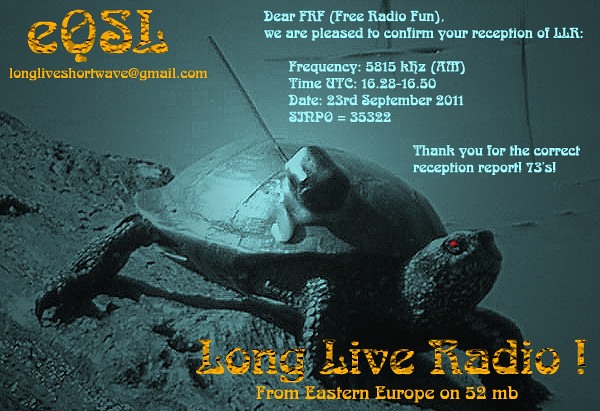This is a vibrant, colored postcard-like advertisement prominently featuring a turtle standing on a rocky surface in the center of the image. The postcard, likely from a radio station, contains text in various positions around the turtle. In the upper left corner, it reads "EQSL: longliveshortwave@gmail.com." Below this, a message addresses "Dear FRF" (Free Radio Fun) and confirms the reception of LLR (Long Live Radio) on a frequency of 52 MB. Additional text includes "We are pleased to confirm your reception of LLR," indicating it as a confirmation of reception report, and a closure with "73," a common ham radio sign-off meaning "best regards." The colors within the image include orange, gray, green, light blue, red, and black, which add to the engaging visual appeal of this unique and specific piece of radio advertising from Eastern Europe.